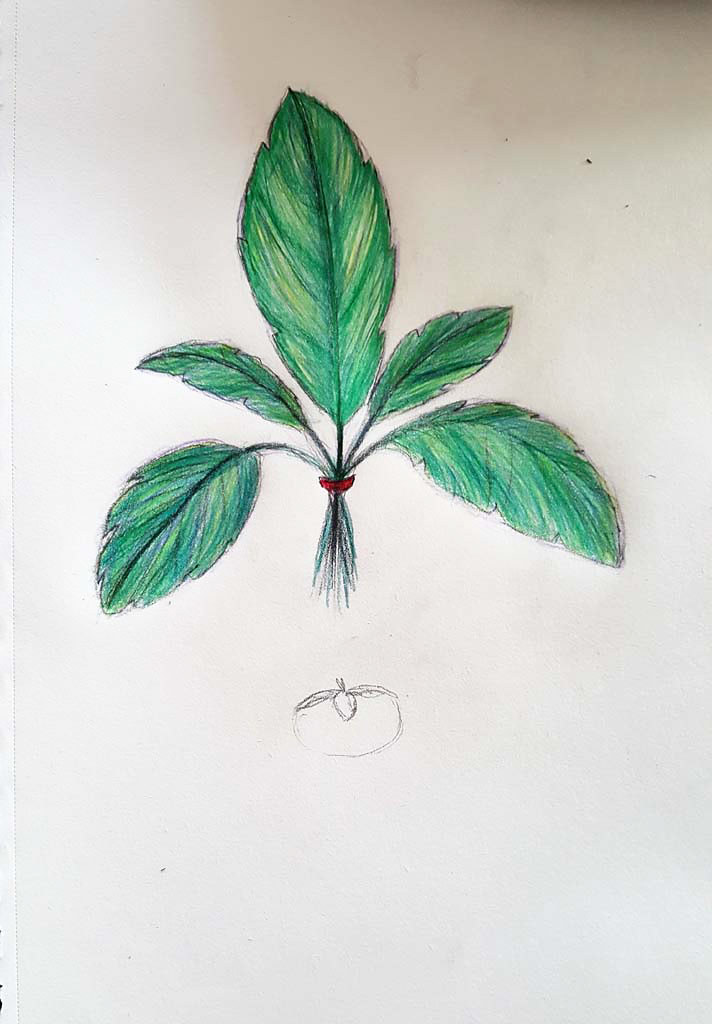This is an intricate hand-drawn image created with colored pencils and crayons on plain white paper. The artwork features a vibrant arrangement of five green leaves, varied in size but uniform in shape, meticulously shaded to show depth and texture. The leaves are bundled together with a distinct red elastic band, creating a fan-like bouquet. The central leaf stands tall and vertical, flanked by two narrow leaves in the middle, and framed by two larger, drooping leaves at the bottom. Each leaf displays detailed veins and stems that seamlessly converge at the red elastic. Below this vivid arrangement, an unfinished pencil sketch hints at what could be a tomato or a peach, providing an intriguing contrast to the vivid green leaves above.